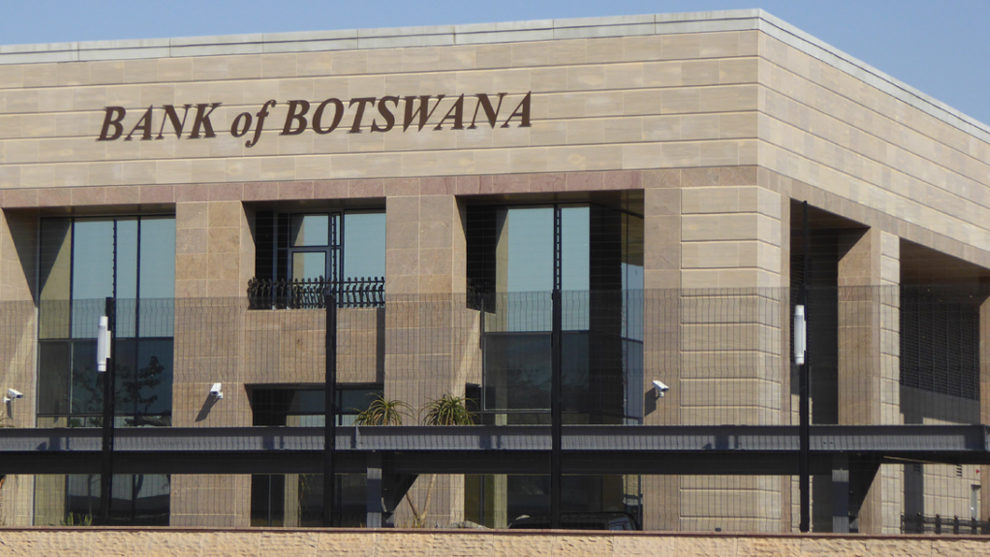This photograph captures the front façade of the Bank of Botswana, a two-story rectangular building constructed primarily of light grey and tan stone with some brick elements. Dominating the image, the bank extends horizontally almost the full width of the frame, with a clear, light blue sky visible in the upper right corner. Across the top of the building, large, italicized letters in a dark brown shade spell out "BANK OF BOTSWANA," with "BANK" and "BOTSWANA" fully capitalized and "of" in lowercase.

The front of the building is characterized by a series of vertical windows divided by stone columns, their reflective surfaces appearing black with a hint of reflection. Below these windows, the photograph shows the top of a security fence that runs in front of the building, consisting of a tall metal framework and mesh panels. Additionally, a small palm tree, splitting into two fronds, is visible in front of the building behind this fence.

The structure's entrance is situated on the front side, flanked by security cameras mounted on the left and right corners. A portion of textured brick, likely part of a wall or additional fencing, is seen at the very bottom of the image, distinct from the stone of the building itself. The photograph neatly encapsulates the prestigious and secure atmosphere of the Bank of Botswana, enhanced by its clear, uncluttered architectural lines set against a serene sky.